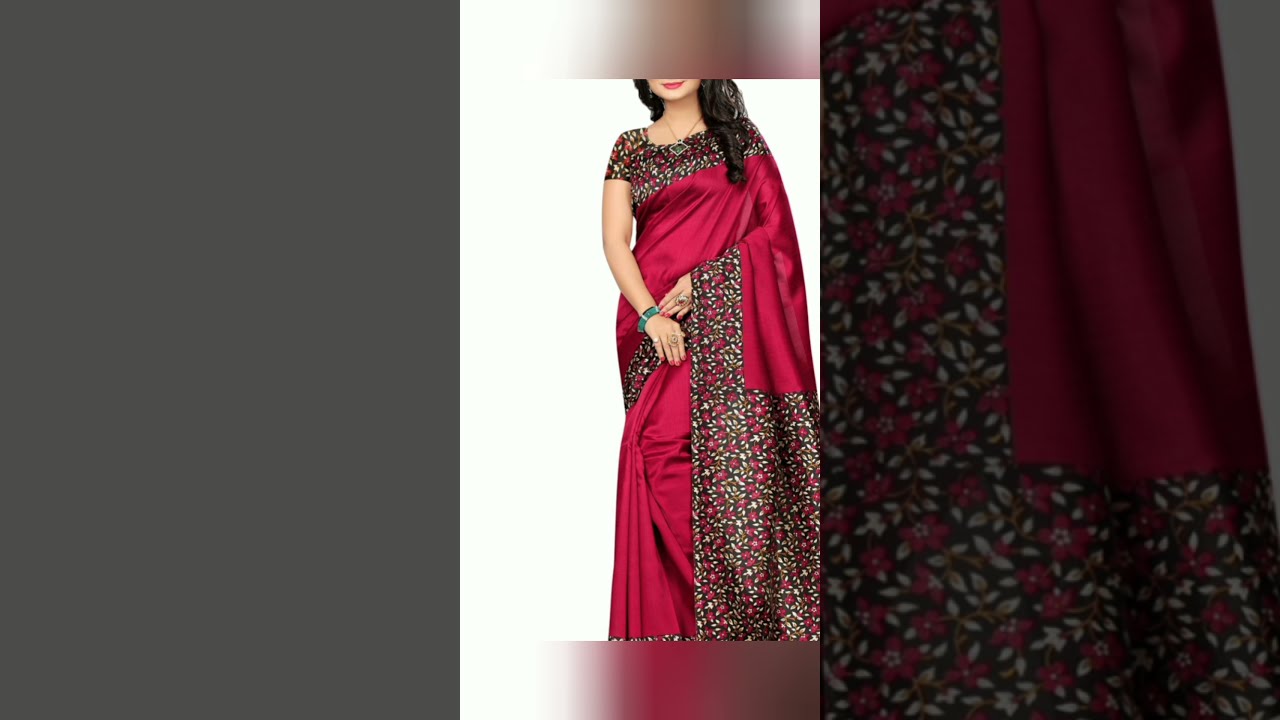The image depicts a woman dressed in a traditional, floor-length, maroon Indian dress adorned with intricate floral patterns. The dress features ornate black trims with fuchsia flowers, green stems, and leaves. Her dark black hair is curled and cascades past her shoulders, complementing her caramel-colored skin. The dress's top part showcases black, white, and red flowers, continuing down to her stomach and arms.

The photo is vertically oriented, with gray or blacked-out sides and a blurred gray top and bottom, obscuring her face above the lips and the lower part of the dress. She wears a gold necklace with a charm, multiple rings on both hands, a blue watch, and a green bracelet. Her lips are painted in maroonish-red lipstick, matching her meticulously manicured nails. The background is stark white, and the woman stands slightly to the right side of the image, emphasizing the focus on her fashion-forward attire and accessory details.